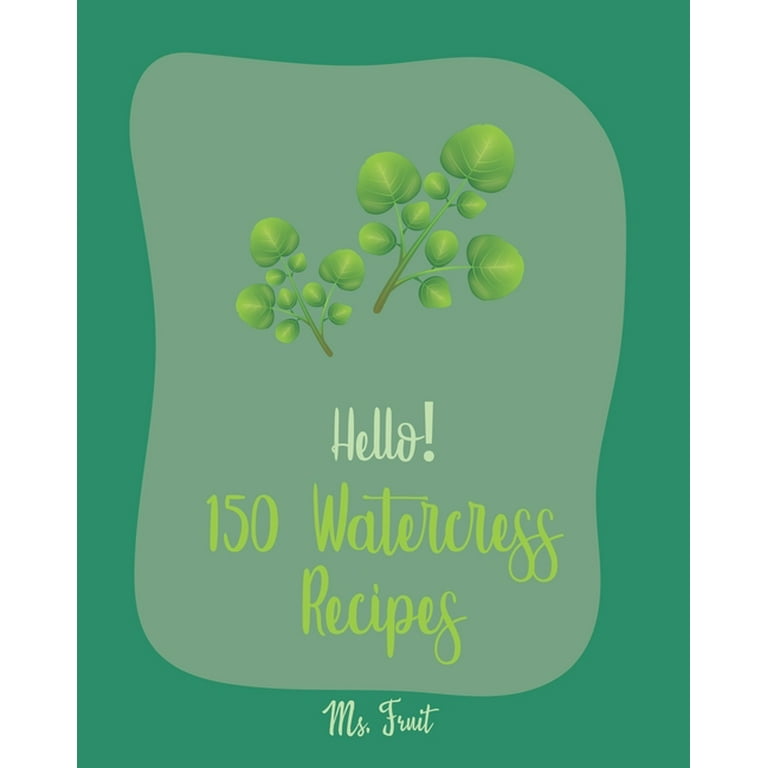This image appears to be the cover of a recipe book, likely titled "150 Watercress Recipes" by Ms. Fruit. The cover features a vertical rectangular shape with a green background, overlaid by a wavy, grayish-green blob occupying the central portion. At the top, two artistically drawn branches with round green leaves extend, one toward the top left and the other toward the top right. Below these branches, in a pale gray script, the word "hello!" is written. Following this, in pale green script, the title "150 Watercress Recipes" is centered. At the bottom of the image, also in pale green script, the author's name, "Ms. Fruit," is displayed. This simple yet elegant design highlights the natural theme of the book with its minimalist artwork and harmonious color palette.